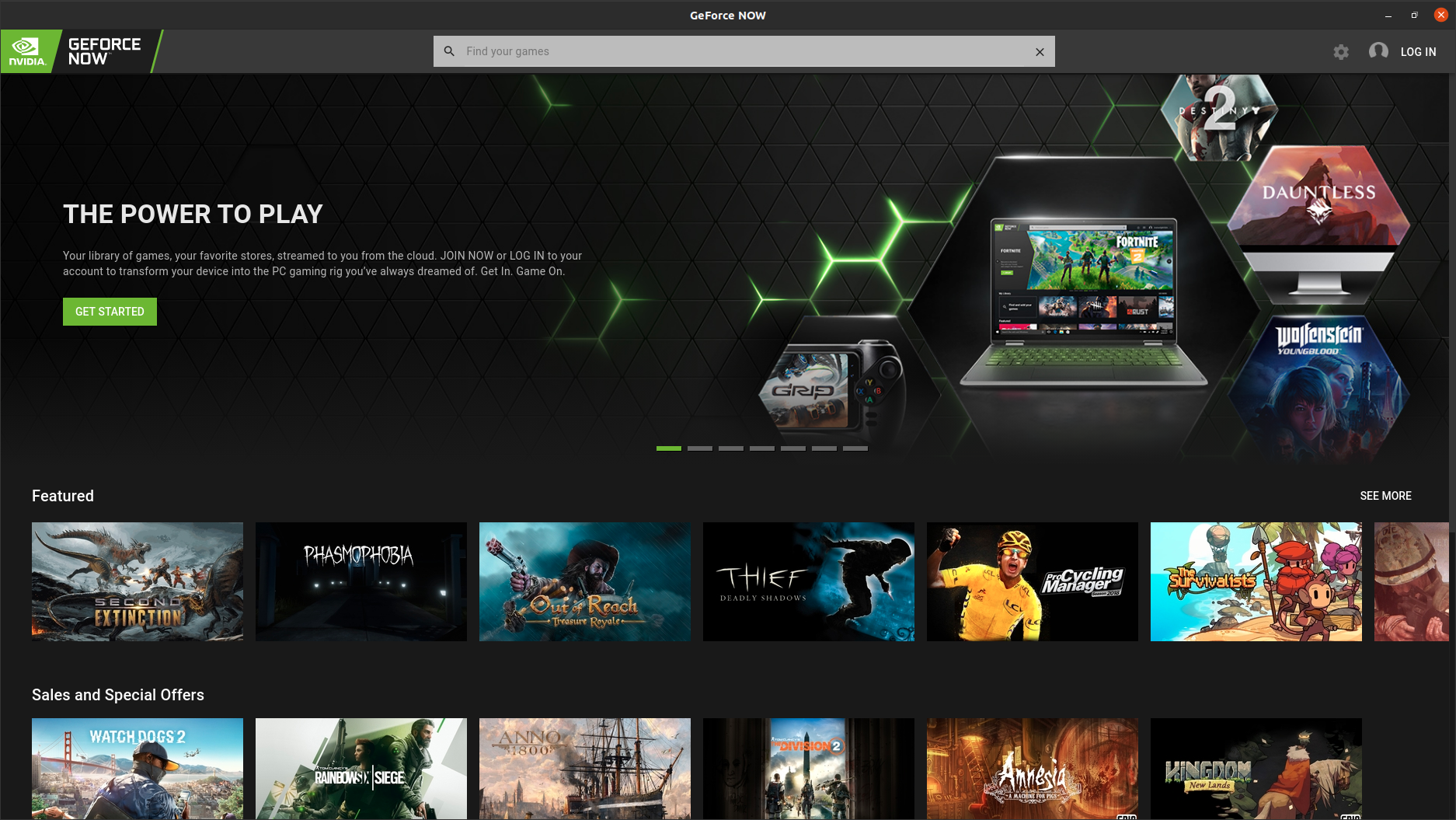This screenshot captures a desktop or laptop running a Linux-based operating system, likely Ubuntu, as suggested by the customized GNOME session visible through the user interface with close, minimize, and maximize buttons at the top of the window. The active window is titled "GeForce Now," and the interface prominently features the GeForce Now logo and name, incorporating the iconic NVIDIA 'eye' logo within a square.

To the right of the GeForce Now title and logo, there's a search field, followed by a settings button and a login button. Immediately below these elements is a scrolling banner advertisement with the slogan: "The Power to Play. Your library of games, your favorite stores streamed to you from the cloud. Join now or log into your account to transform your device into the PC gaming rig you've always dreamed of. Get in, game on." This promotional message is encouraging users to either sign up or log in to access the cloud gaming service.

A bold, green "Get Started" button with white text stands out below the banner, inviting users to begin their gaming journey. Additionally, the screenshot showcases various game thumbnails available on the service, including titles like Dauntless, Destiny 2, Wolfenstein, and GRID. Further down, there’s a section highlighting featured games such as Phasmophobia, Out of Reach, Thief, and Cycling Manager, demonstrating the diverse gaming options supported by GeForce Now.